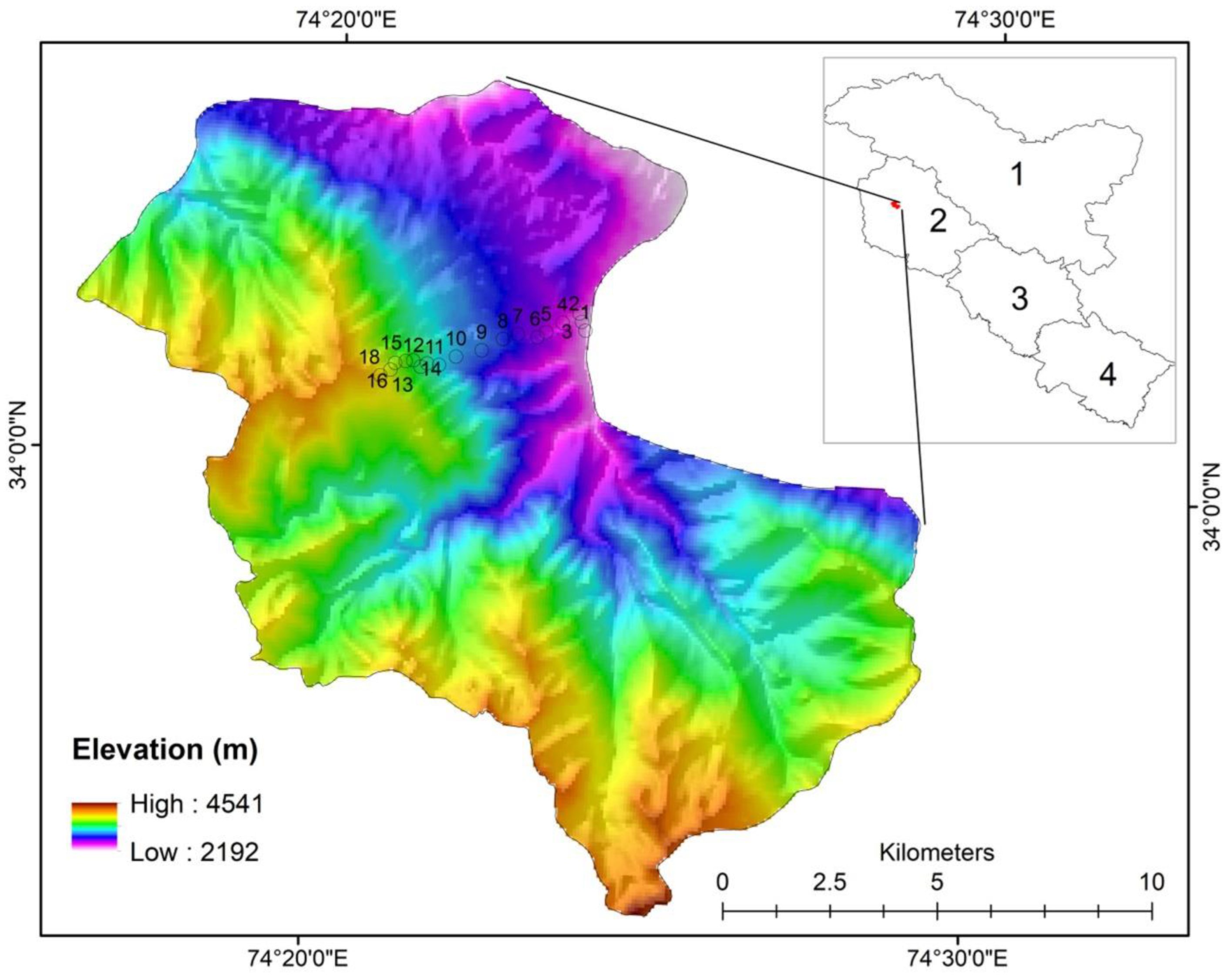The image is a detailed color-coded elevation map framed by a black border forming a square. The upper left-hand corner features a gray box with three labeled sections numbered 1 through 4, where section 2 contains a distinct red dot with arrows pointing towards the main map. The map itself illustrates an unidentified landmass, possibly an island, segmented into different regions with a gradient elevation scale ranging from high in red (4,541 feet) to low in purple (2,192 feet). Colors such as purple, blue, green, yellow, and orange represent various elevations, with green likely indicating lower elevations and gold, higher terrains or sandy areas. The lower left corner displays an elevation key that shows this gradient from purple to red, labeled with the letter 'M' for meters. The lower right-hand corner includes a gauge that interprets the scale of the map in kilometers per inch. The borders of the map are marked with longitude and latitude coordinates, indicating precise geographical positioning.